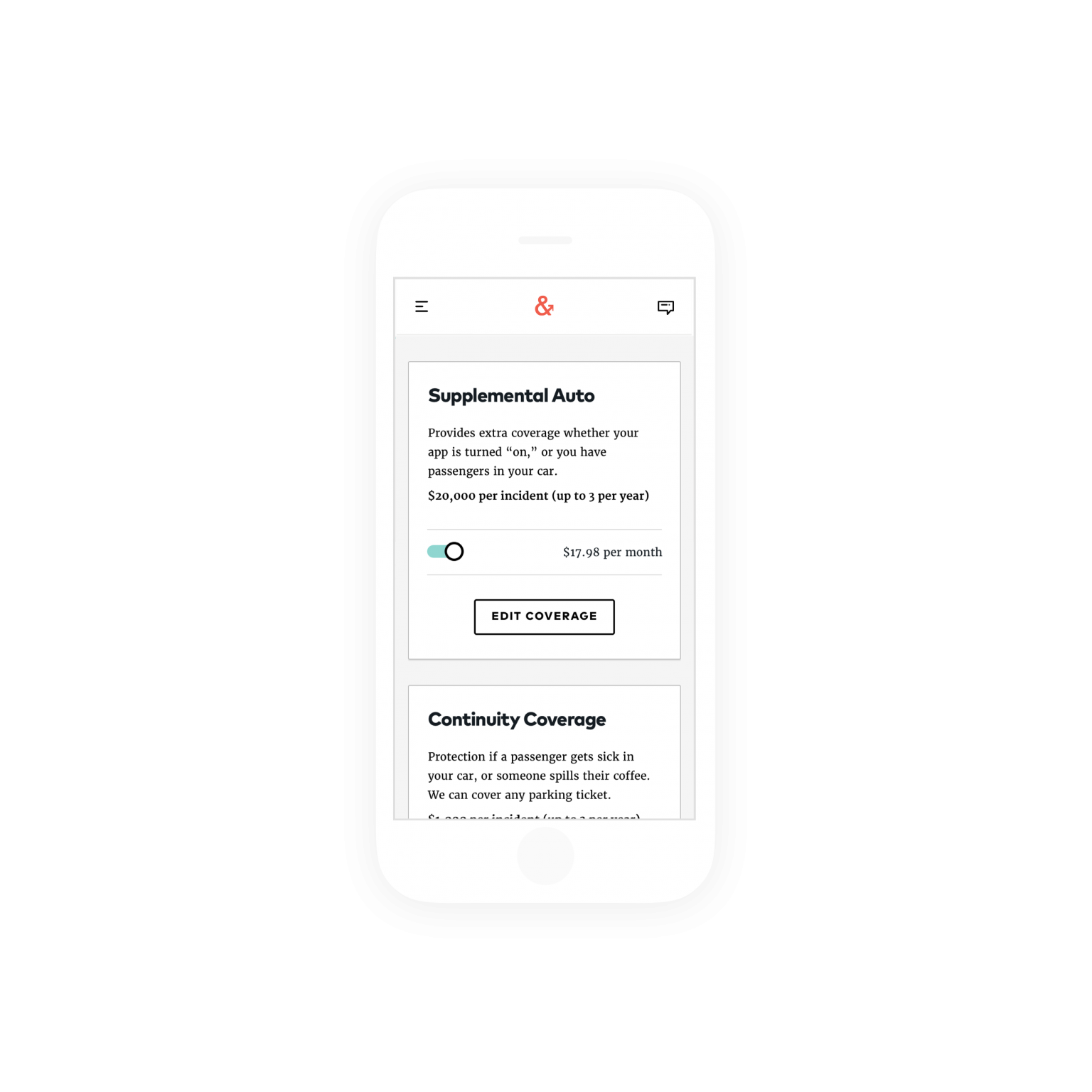In the image, there's a white smartphone displaying an insurance application. At the top left of the screen, there's an icon with three horizontal lines, often used as a menu button. Positioned centrally at the top, there is a red icon featuring an ‘&’ symbol with a small arrow. On the top right, an icon representing subtitles or captions is visible.

Moving to the middle section of the phone’s screen, there’s a large white text box. Inside, in bold black letters, it reads "Supplemental Auto." Below this, smaller text explains the coverage details: "Provides extra coverage, whether your app is turned on or you have a passenger in the car. $20,000 per incident, up to three per year." Adjacent to this, there is an option to select or deselect this coverage, which is priced at $17.98 per month. A button labeled "Edit Coverage" allows further customization.

Towards the bottom of the screen, part of a second text box is visible. The prominent text reads "Continuing Coverage," while the smaller text beneath it explains: "Protection if a passenger gets sick in your car or someone spills their coffee. We can cover any parking ticket." The remaining text is cut off and not fully visible on the screen.